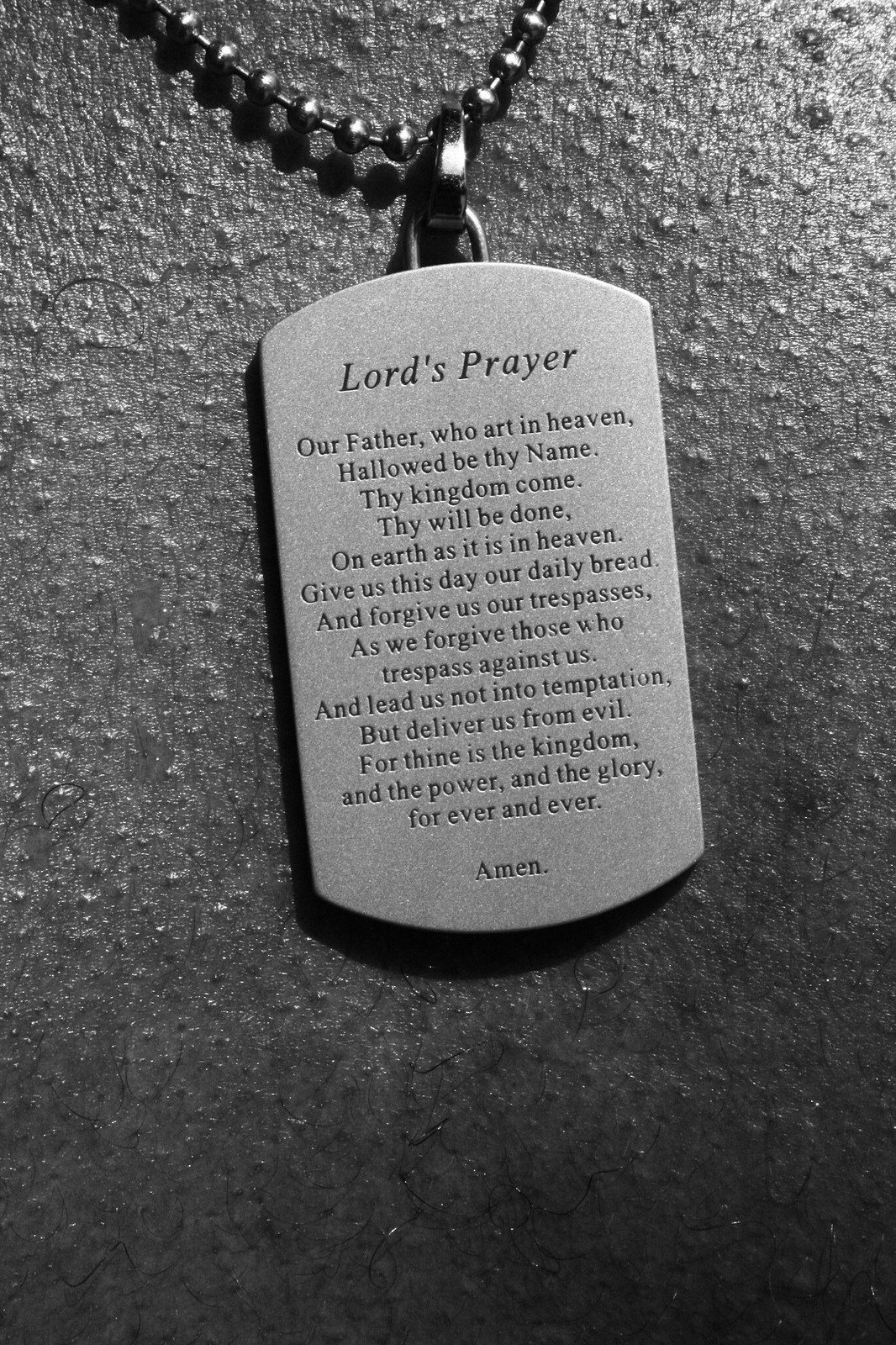This is a tall, rectangular black and white photograph of a necklace resting against a silvery, bumpy textured background that appears to be human skin with small black hairs protruding from it. The image features a silver string necklace visible at the top left corner, consisting of evenly spaced silver spheres. The light reflects off the top of the skin, growing darker and grayer toward the bottom right corner. Attached to the necklace’s clasp is a gray pendant, shaped like a vertical rectangle with a curved top and bottom. The pendant is engraved with the Lord's Prayer in a center-justified, larger font at the top reading "Lord's Prayer," followed by the full text of the prayer in smaller font. The engraved text reads: "Our Father who art in heaven, hallowed be thy name, thy kingdom come, thy will be done on earth as it is in heaven. Give us this day our daily bread and forgive us our trespasses as we forgive those who trespass against us and lead us not into temptation, but deliver us from evil. For thine is the kingdom and the power and the glory forever and ever. Amen."